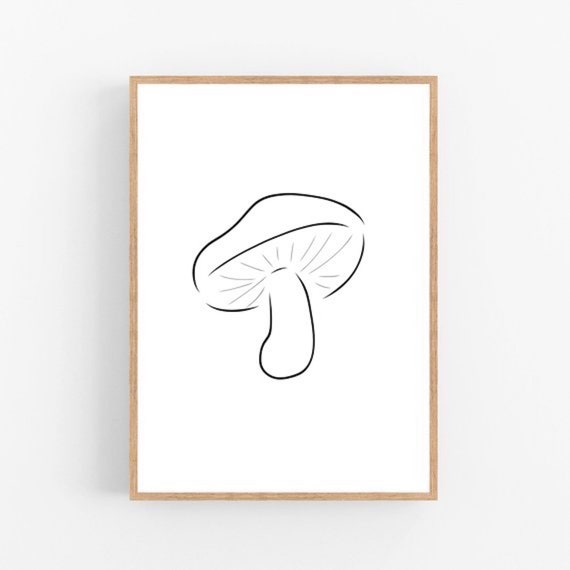The picture is a simple, black ink drawing of a mushroom, centered on a white canvas. The mushroom is depicted as a silhouette with minimal detail, primarily on the lower end, showing a thick stem and lines suggesting the underside of the cap. The mushroom outline is slightly tilted backwards and occupies about half of the canvas. The artwork is framed in a wooden frame, which is predominantly light-colored with some slightly darker patches. The frame, which encompasses the entire rectangular picture, is set against a white background and casts a slight shadow to the left side.